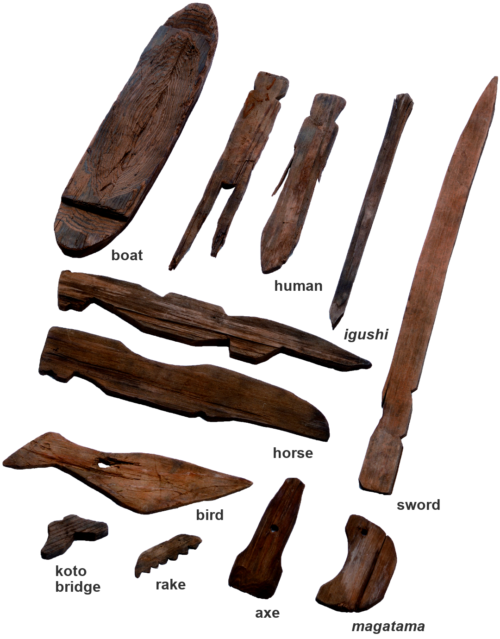The image showcases a collection of primitive tools and artifacts, seemingly used by an ancient civilization, displayed by an Archaeological Association. These objects, which appear to be either wooden or fossilized, are each carefully labeled. At the bottom, we have items like "Koto Bridge," resembling two small wooden pieces shaped like jelly beans, and a comb-like artifact labeled "rake." Next to these, we see an "axe," a "magatama" stone, all of which are equally primitive in appearance. Moving up, there is an object labeled "bird," which is misleadingly a flat piece of wood. Above this is an item marked as "horse," which too appears as an unrefined wooden piece. A sword-like wooden piece sits on the right side, labeled appropriately as "sword." At the topmost row, arranged diagonally, are items labeled "boat," shaped like a small surfboard, a thin piece marked "human," and another mysterious object tagged "Igushi." Despite some confusion over the exact nature and origin of these objects, they are evocative of ancient Japanese culture and highlight the rudimentary craftsmanship of early civilizations.